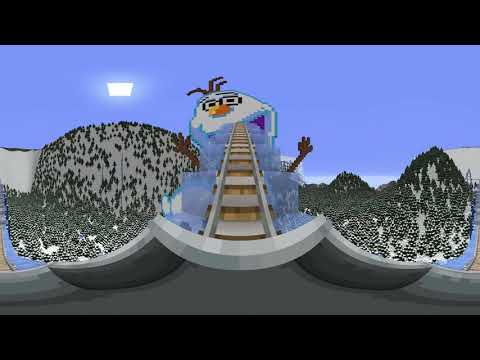The digital artwork presents a whimsical and detailed scene within a wide rectangular format, bordered by thick black rectangles at the top and bottom. Dominating the upper half of the image is a light purple background, with a shining white square positioned at the top left corner, adding a luminous touch. Central to the composition is a cartoonish figure resembling a snowman, characterized by a circular white face, an orange nose, and three distinctive tufts of hair sprouting from its head. The snowman's mouth is open wide, extending downwards where it morphs into a gray and brown railroad track that runs towards the bottom of the image. Framing this surreal scene, a dense forest of large, dark green trees, heavily laden with snow, stretches out on either side of the tracks. Notably, the bottom of the image features a curved shape, adding to the fantastical milieu. The color palette spans from the brightness of white and light purple to the earthy tones of brown and green, contributing to the overall vivid, animated, and dream-like setting.